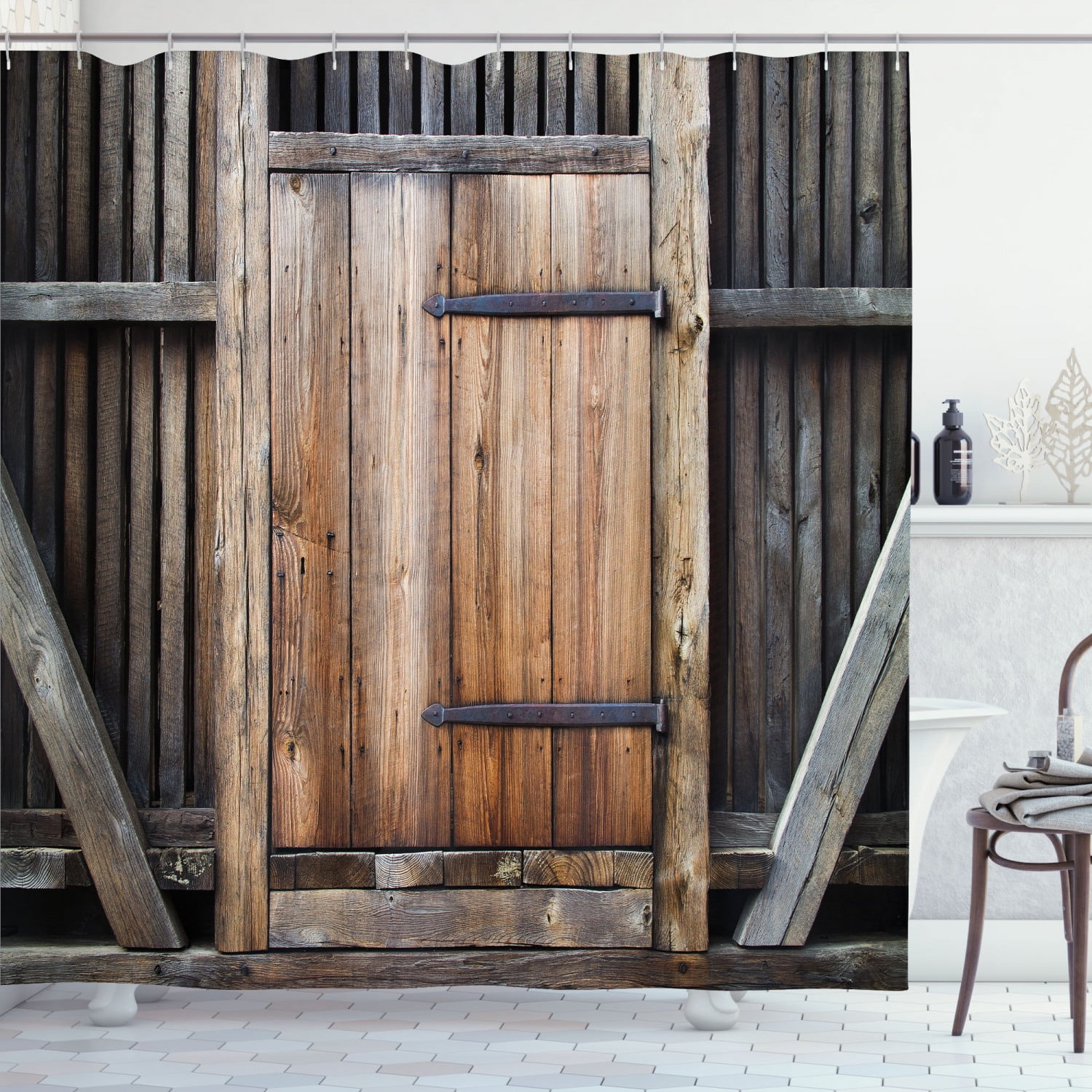The image depicts a staged and heavily edited photograph of a square-shaped bathroom scene. The focal point is a clawfoot tub made of white porcelain resting on a floor of white hexagonal tiles. Next to the tub is a brown metal chair with a gray fabric draped over it. In the background, a small gray wall with a white ledge displays a bottle of soap and metal carved leaf statuettes. Running horizontally from the top left to the right edge of the image is a gray shower curtain, suspended by multiple gray rings. The shower curtain features a highly realistic, but clearly edited, depiction of an old barn door. This faux barn door design includes weathered wood, large metal hinges, and angled wood pieces, adding an intricate rustic element to the scene. To the right of the curtain, the bottle of soap with a black pump top and other small knickknacks are clearly visible on the ledge. The overall ambiance is a blend of vintage charm and modern staging.